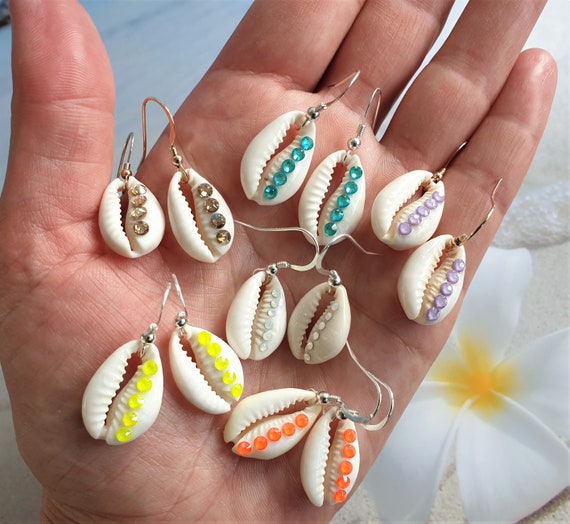A close-up photograph captures a fair-skinned hand, palm up, displaying six pairs of tiny seashell earrings. Each pair of white oval shells, featuring teeth-like openings, is affixed with assorted colored gemstones along the right side in a vertical alignment. The gemstones include shades of translucent brown, turquoise blue, lilac purple, bright white, vivid orange, and a yellow-green hue. The earrings are attached with French hook findings in brass, gold, and silver tones. In the background, a white plumeria flower with yellow accents appears alongside hints of ocean and sand, suggesting a beach setting. The image, resembling an Instagram post, likely serves to advertise the handmade seashell earrings for sale.